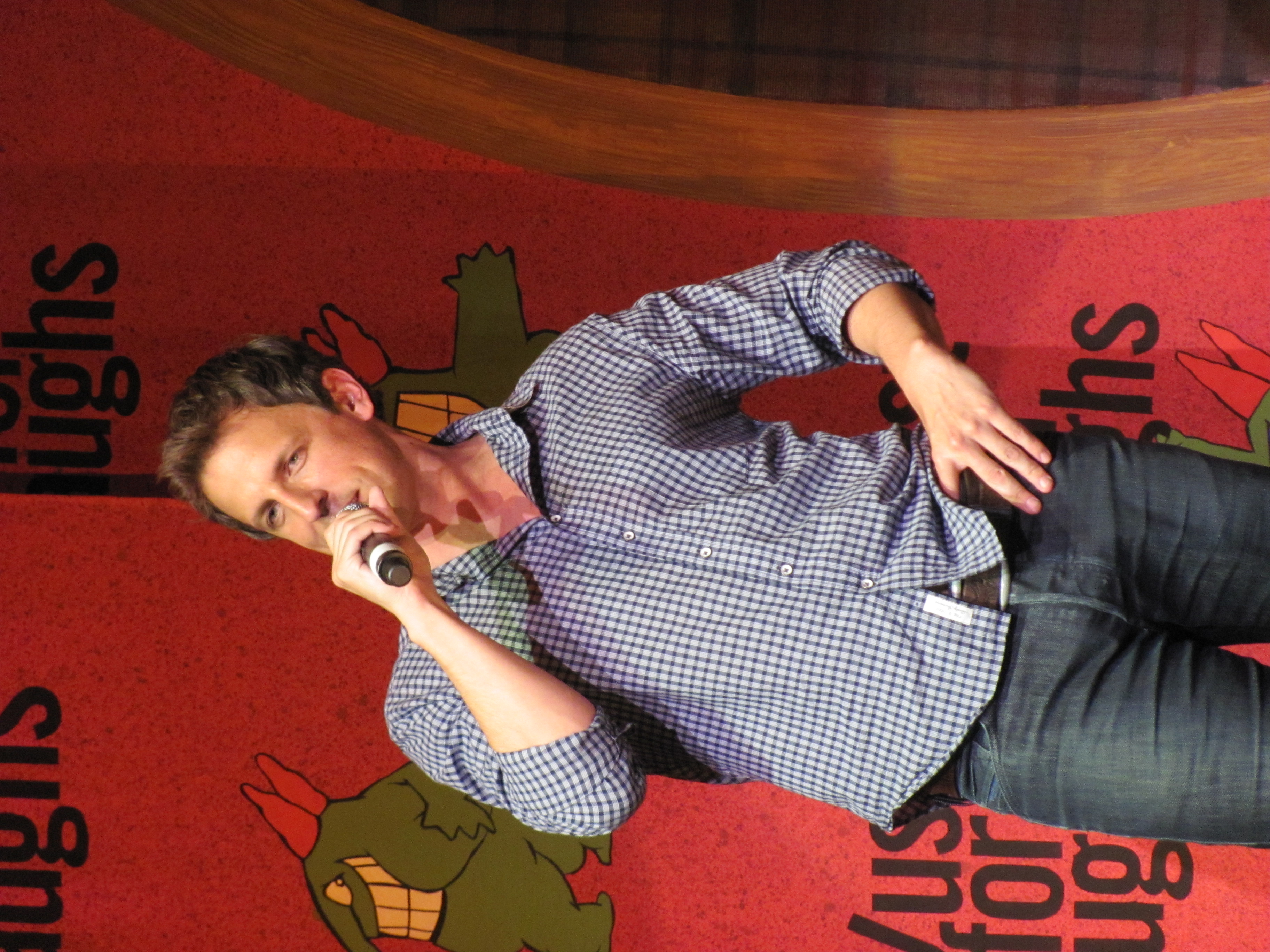In this sideways photo, a man who resembles Seth Meyers, stands before an audience, gripping a black microphone with a white strip near its base in his right hand, while his left hand rests on his waist. He wears a plaid blue and white long-sleeved shirt, slightly rolled up, blue jeans held by a dark belt with a silver buckle, and brown hair visible on the left side. The backdrop, prominent in the shot, features a red wall adorned with several green, horned creatures sporting big smiles and white teeth. Black letters, partially obscured by the man, spell out words like "LAS," "US," and "FOR." A brown wooden frame outlines a plaid or checkered pattern at the top, in hues of white, blue, and red.